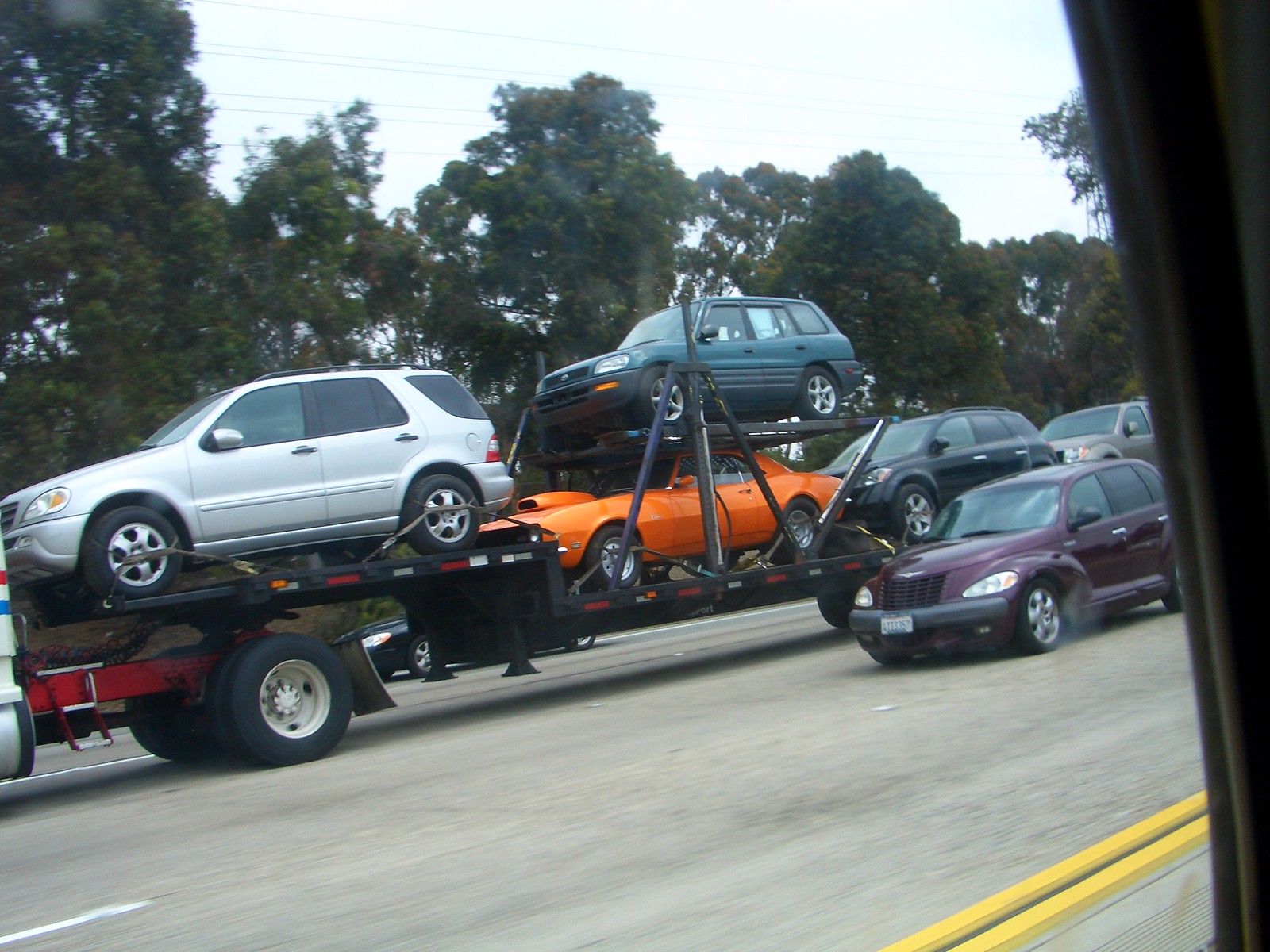The photograph captures a highway scene in motion, taken from inside a moving vehicle. At the center of the image is a trailer of a large semi-truck, which is hauling multiple stacked cars. There are up to six cars on the trailer, with a grey Mercedes SUV at the front, followed by a green SUV, likely a Subaru, on the top. Below the green SUV is an orange muscle car distinguished by its large headers. Behind this muscle car is a dark blue vehicle, and further back, two more silver cars are visible. The image, which seems to have been taken in the late 1990s, features additional elements such as tall trees lining the road, power lines in the background, and yellow road divider lines in the front right corner. To the right of the truck, a purple car, possibly a PT Cruiser, can be seen slightly more in the foreground on the busy, wide road.